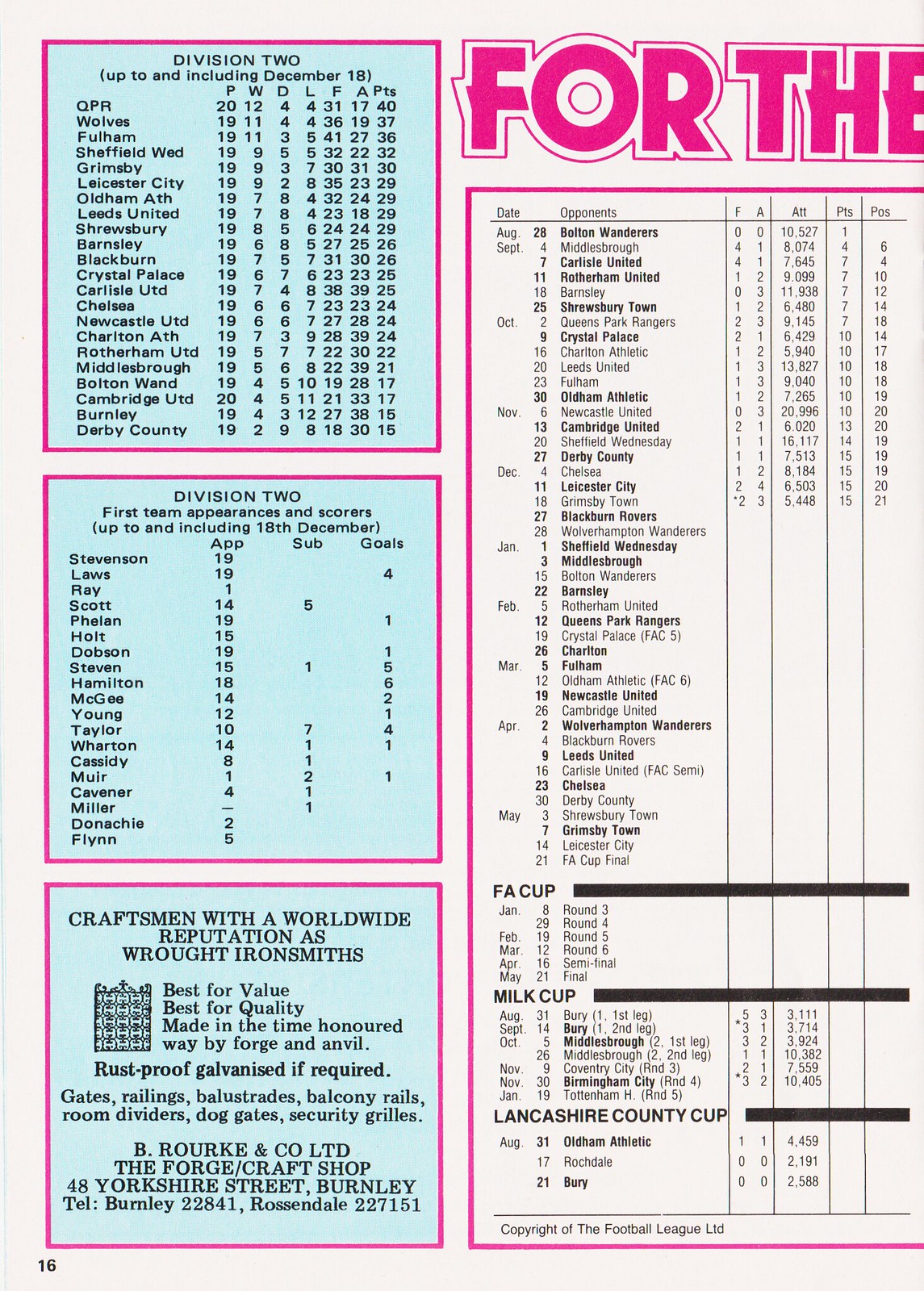This detailed photograph captures a slightly cut-off page, predominantly covered in text organized into distinct blue boxes with pink borders and a central white box with pink borders. The top title is not fully visible, revealing only "For the." The main content pertains to English Football League Division 2, listing team names such as QPR, Wolves, Fulham, Leicester City, Oldham Athletic, Leeds United, and several others, offering details up to and including December 18th. This suggests the image could be from a sports magazine or a listing relevant to a certain period. Additionally, there’s a section advertising Bergens Limited, renowned craftsmen in wrought ironwork, detailing their offerings: gates, railings, balcony rails, and more, with their shop based at 48 Yorkshire Street, Burnley. The visual composition incorporates colors like tan, purple, light blue, black, white, and gray, mostly occupying the entirety of the image, lending to a historical and informative feel.